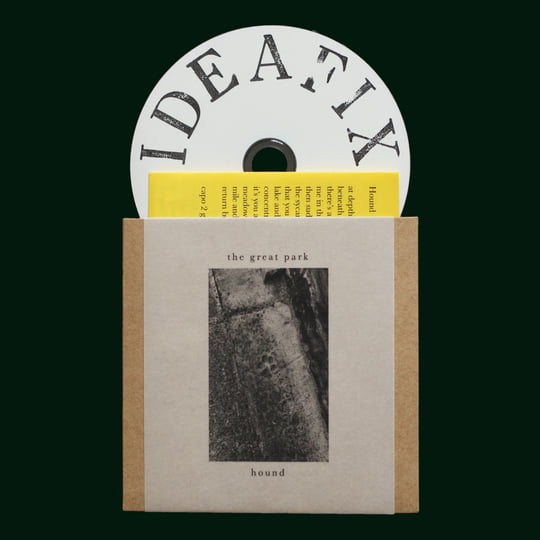The advertisement features a video disc or CD partially emerging from its light brown and off-white package. The package displays the album or video titled "The Great Park" by an artist named Hound, with all text in lowercase. The disc itself is white with black, crudely printed letters that read "Idea Fix" or "Idea Fice," the exact wording unclear. The cover art showcases a paw print on a concrete street, further reinforcing the theme of the package. The overall design is minimalistic, with a focus on the artist’s name, album title, and the striking paw print image.